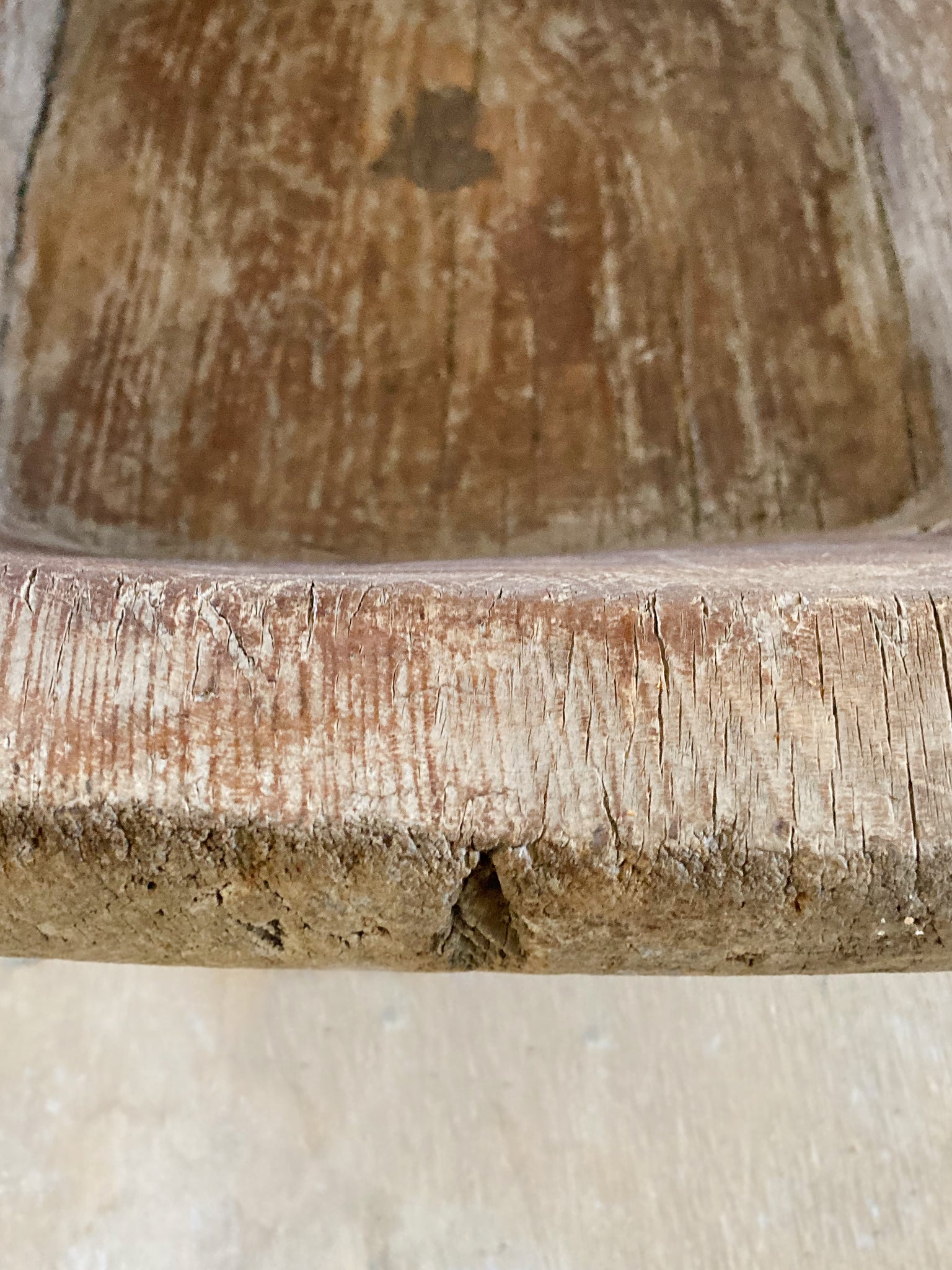The image captures a close-up of an aged and severely weathered wooden board that occupies the majority of the frame, approximately 90% of the image. The wood shows a cross-section, revealing its thickness and part of its length. It is dominated by different shades of brown, with patches of a whitish-gray background peeking through. The board appears to have once been stained or varnished, but this finish has largely worn away, exposing the natural wood grain beneath. The wood is visibly dry and cracked due to prolonged exposure and lack of protective coating. A prominent feature is a hole on the bottom side, possibly resulting from rot or insect habitation. The edges of the wood are slightly rounded, adding to its rustic appearance. Overall, the photo has a monotone composition with a creamy, blank background that contrasts with the texture-rich wood.